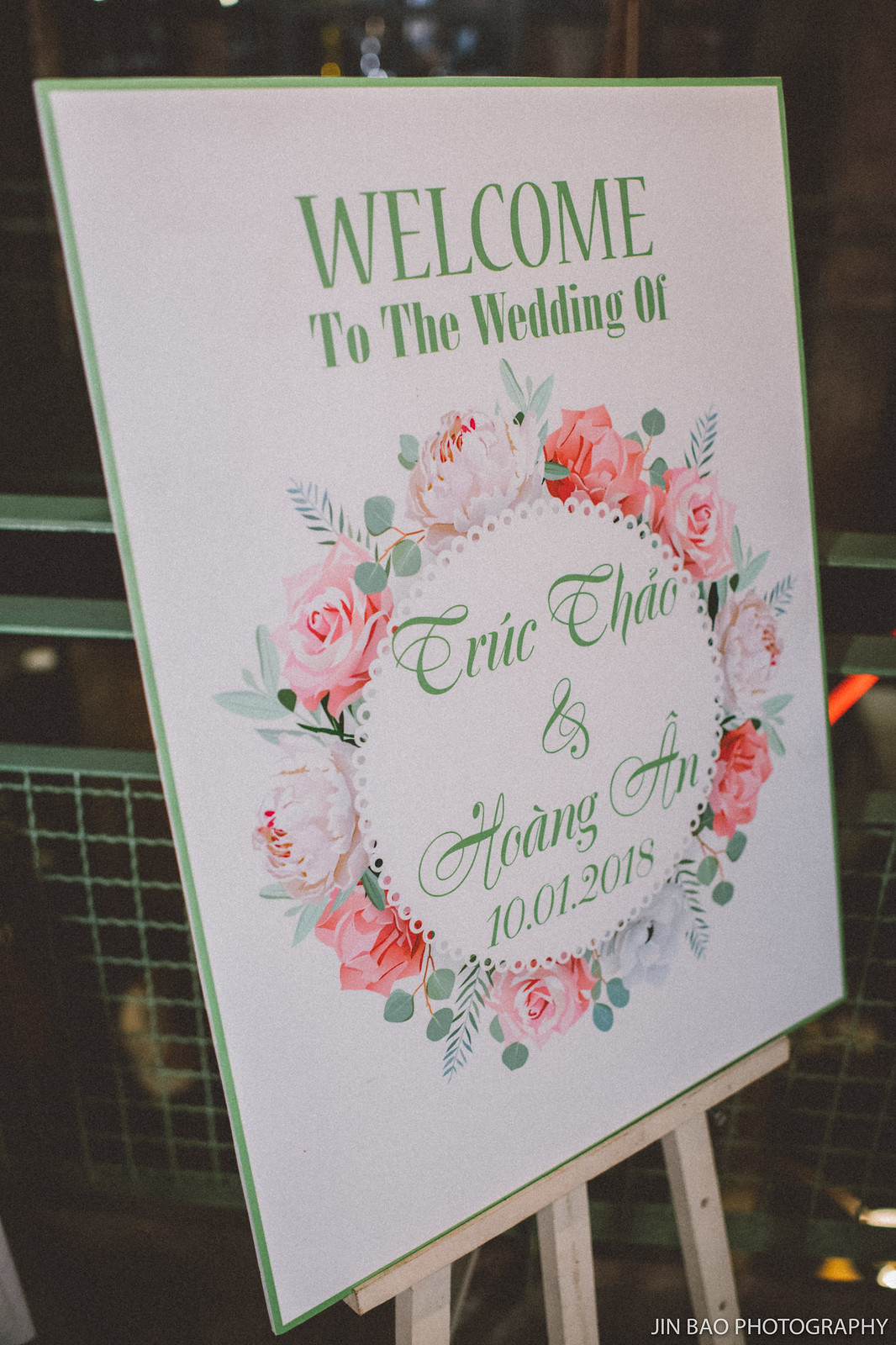This image captures an elegant wedding welcome sign displayed on a wooden easel. The sign, with a pristine white background and a mint green border, warmly greets guests with the words "Welcome to the wedding of" in an ornate, green font. Central to the sign is a circular floral wreath composed of red, bright pink, and light pink roses intertwined with lush green leaves and ferns. Inside this delicate wreath, the names "Truc Chau and Hoang An" are inscribed, albeit in a challenging-to-read font, alongside the date "10-01-2018." The backdrop of the image features a metallic fence and some open ground. At the bottom right corner, a watermark reads "Jin Bao Photography," confirming the image's professional capture. This picturesque sign ensures guests know they have arrived at the wedding venue, though it provides no additional venue details. The blend of green, pink, and white hues gives the sign a fresh, spring-like ambiance.